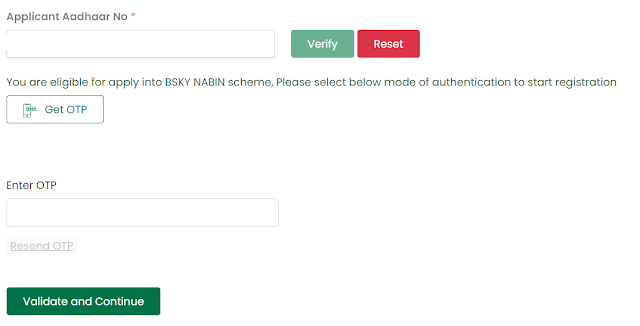**Detailed Caption for Image:**

The image depicts a form for applying to the "BSKY NABIN scheme," presumably accessible on a website, though no specific website details are shown. In the upper left corner, there is a label "Applicant AADHAAR NO," written in black with a red asterisk above the "NO" indicating a mandatory field. Beneath this label is a white rectangular input field for entering the Aadhaar number. Adjacent to this input field, on the right side, there are two buttons: a green rectangle labeled "Verify" and a red rectangle labeled "Reset."

Below these fields, there is an instructional text stating: "You are eligible to apply to the BSKY NABIN scheme. Please select below mode of Authentication to Start Registration." Directly below this instruction is another white rectangular field accompanied by a drawing of a cell phone, likely indicating a method to receive a One-Time Password (OTP). 

Following this, there are the words "Enter OTP" above another white rectangular input field where the received OTP can be entered. Beneath this field, there is a clickable link reading "Resend OTP" for users to request a new OTP if needed. Finally, at the very bottom of the form, there is a large green rectangle with the text "Validate and Continue" in white letters, presumably to proceed with the registration process after entering the required information.